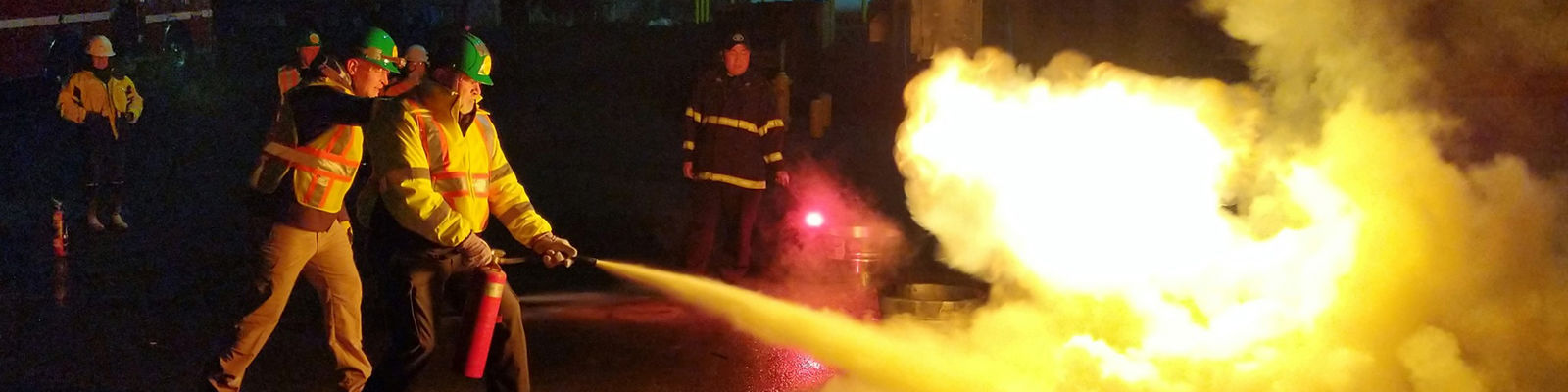The image, a narrow horizontal nighttime shot, vividly captures a team of firefighters actively battling a fire. In the foreground, an older firefighter, clad in a yellow jacket with orange and darker stripes, dark pants, and a green protective helmet, is seen spraying flames with a fire extinguisher. His determined focus contrasts with the surrounding chaos. Directly behind him, another firefighter, wearing similar gear, has a supportive hand on his shoulder, ready to assist. To the right, another man, distinguishable by his black jacket with yellow stripes, also stands guard. The background reveals several more firefighters who, though somewhat obscured by the dim light and smoke, are clearly poised to jump into action. The scene is illuminated primarily by the eerie red and yellow glow of the fire and smoke, casting dramatic, flickering shadows on the courageous first responders. The only additional light sources come from their flashlights pointed into the smoky plume, highlighting their vigilant efforts to contain the blaze.